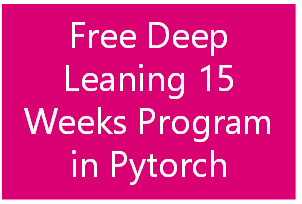The image features a horizontally-oriented rectangular background in a deep pinkish-red color. Centered within this background is a bold, white text spanning four lines that reads: "Free Deep Learning 15 Weeks Program in PyTorch." The text is large and occupies most of the rectangular space, with the line "Weeks Program" being the longest and nearly touching the edges on both sides, leaving only a slight margin. The overall design is minimalist, with the striking contrast between the deep pinkish-red background and the white text making the caption highly legible and attention-grabbing. The mention of "PyTorch" relates to a popular open-source machine learning library, emphasizing the educational nature of the program advertised.